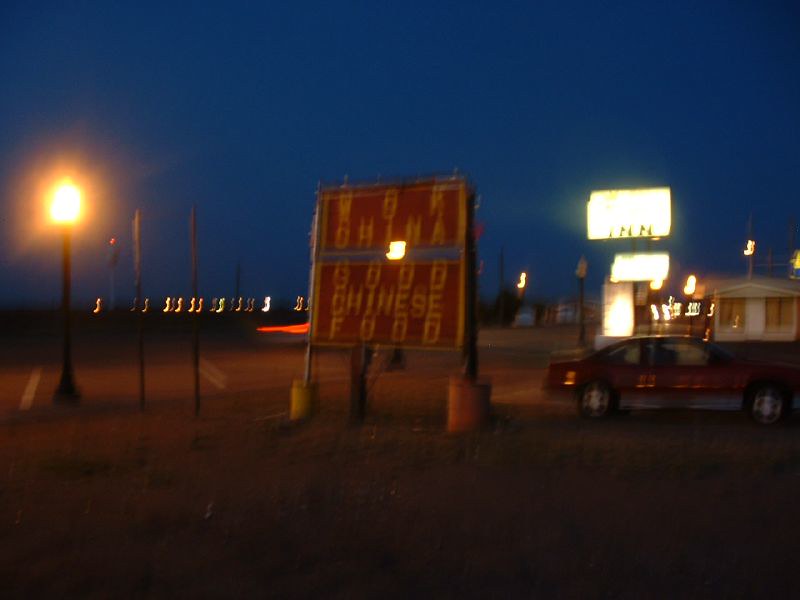This nighttime photograph captures a slightly blurry yet vivid scene under a beautifully deep blue sky, possibly digitally enhanced. Dominating the foreground is a large red sign divided into two rectangles with a white border, advertising "WOK CHINA" and "GOOD Chinese food." The sign is upheld by two cylindrical supports, one yellow and one red, both threaded with metal rods. Below the sign rests a dark gray parking lot, where a maroon sedan is parked to the right.

On the left side of the image, a brightly lit street lamp casts a yellow light, standing in contrast against two additional poles nearby. In the background to the right, an illuminated sign reading "INN" hints at the presence of a motel, albeit with text too blurred to fully decipher. The scene also reveals a small white building and multiple other glowing signs and streetlights scattered in the distance, contributing to the urban nighttime ambiance.